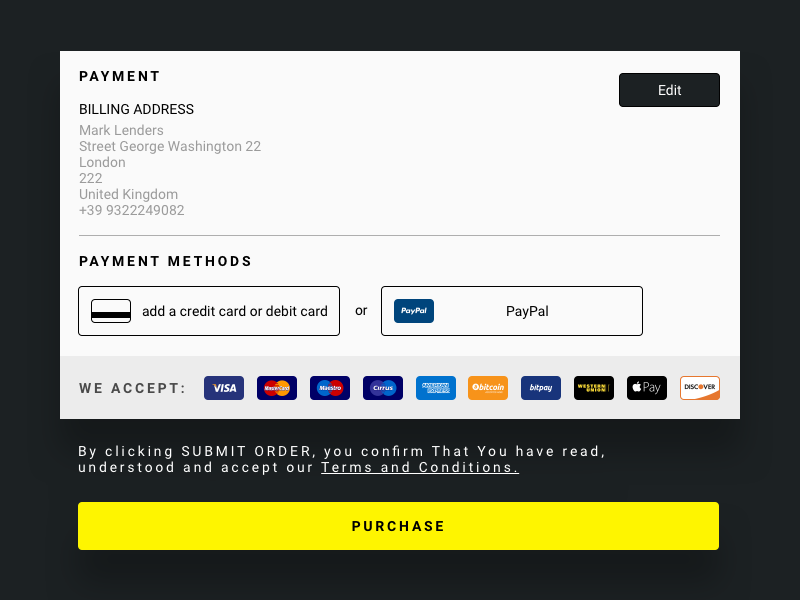In the provided image, a detailed visual interface for an online purchasing platform is displayed. The top left corner prominently features the "Payment" section, while the top right corner presents an "Edit" option. Centrally located is a field labeled "Billing Address" that specifies: "Mark Lander Street, George Washington 22, London 222, United Kingdom," accompanied by a numeric code "39, 93222, 49082." Below this, a horizontal line separates the sections, leading to the "Payment Methods" area. This section includes various icons representing payment options such as credit card or debit card options, and PayPal, envisioned as a square with a stripe through it.

The bottom left corner illustrates the accepted payment methods, listing Visa, MasterCard, American Express, Bitcoin, BitPay, Western Union, Apple Pay, and Discover. A notable piece of text at the bottom specifies, "By clicking Submit Order, you confirm that you have read, understood, and accept our terms and conditions," signaling the final step of the transactional process. This comprehensive layout indicates a well-organized area for inputting billing information and selecting diverse payment methods for completing a purchase.